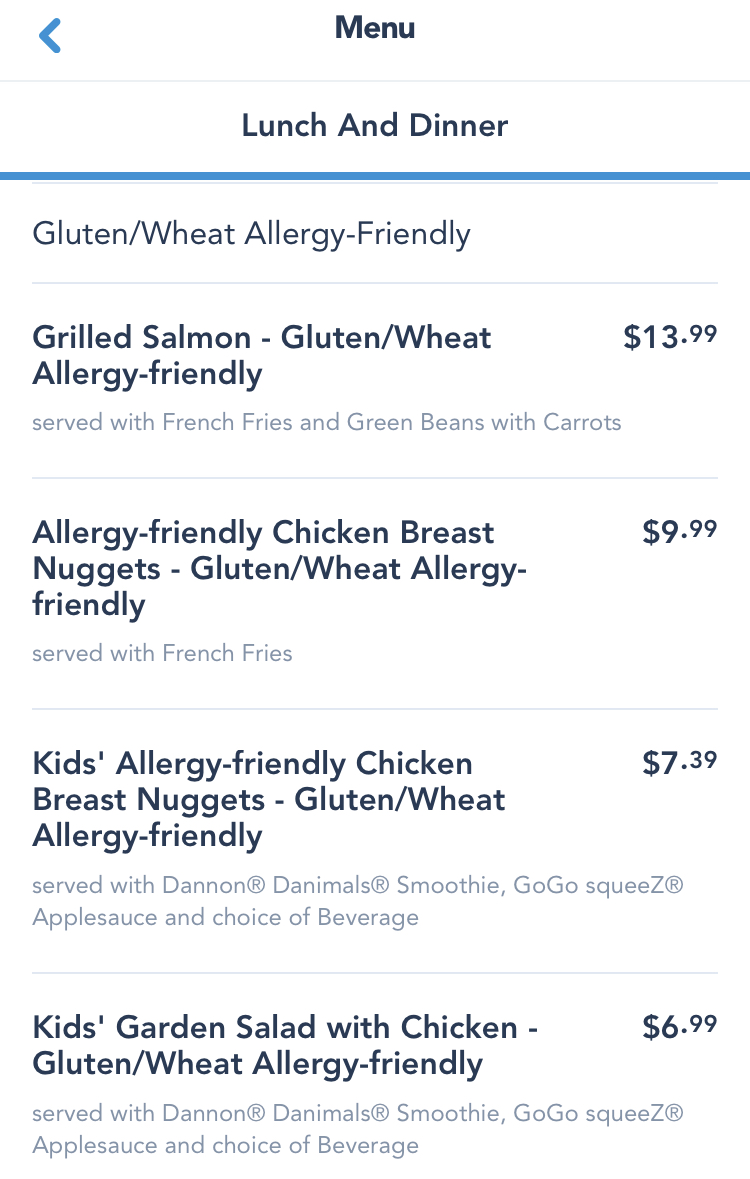This screenshot captures a detailed menu from a dining establishment. At the top center of the image, the word "Menu" is prominently displayed in bold, black text. To the left of the menu title, a blue arrow points left, followed by a light gray horizontal line beneath. Below this, the menu lists offerings for "Lunch and Dinner."

A blue horizontal line separates the title from the items below, which are categorized as "Gluten/Wheat Allergy-Friendly." The items are as follows:

1. **Grilled Salmon (Gluten/Wheat Allergy-Friendly)**: Served with french fries, green beans, and carrots. Priced at $13.99.
2. **Allergy-Friendly Chicken Breast Nuggets (Gluten/Wheat Allergy-Friendly)**: Served with french fries. Priced at $9.99.
3. **Kids Allergy-Friendly Chicken Breast (Gluten/Wheat Allergy-Friendly)**: Comes with Danon Danimals Smoothie, GoGo Squeeze Applesauce, and a choice of beverage. Priced at $7.39.

The menu is designed to cater to those with gluten and wheat allergies, ensuring a safe and enjoyable dining experience for all guests.